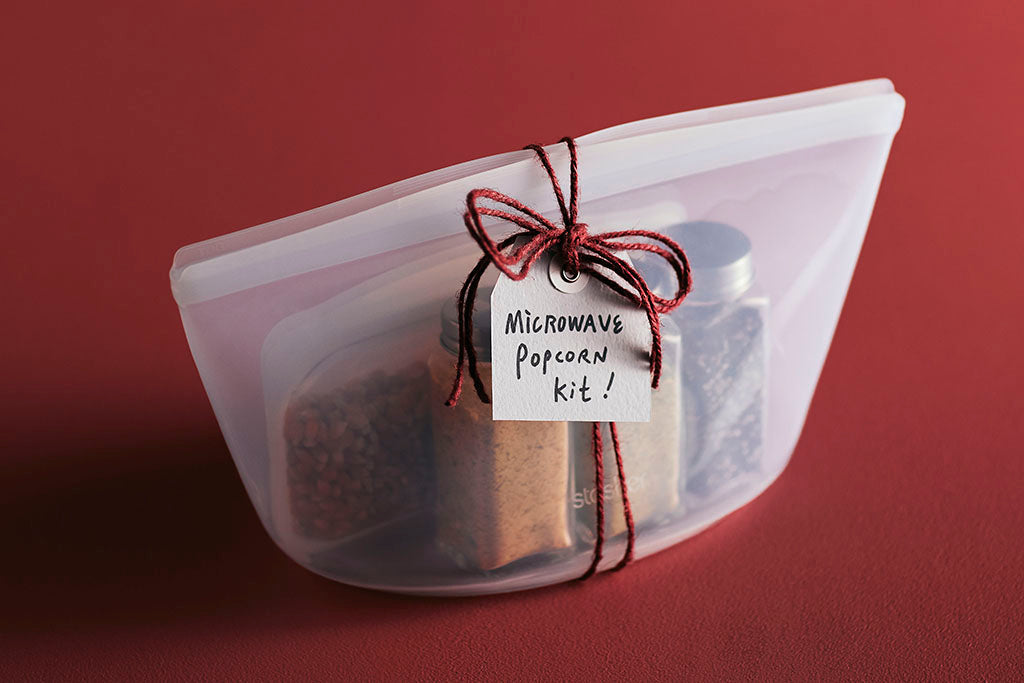A clear, see-through bag labeled "Microwave Popcorn Kit" in bold, black letters is tied with a red string and tagged with a white label. Inside the bag, there is a smaller bag containing popcorn kernels alongside three tall shaker jars of seasonings: one filled with red seasoning powder on the left, a jar of white powder in the middle, and another with black powder on the right. The entire package rests on a textured red table or countertop, with a noticeable shadow cast to the left. The overall presentation is both neat and visually appealing, making it an attractive and practical kit for preparing flavored popcorn at home.